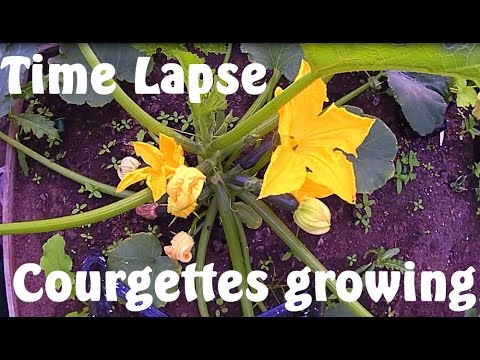The image shows a time-lapse shot of courgettes (likely known as zucchinis in the U.S.) growing in a garden. The central focus is a vibrant plant with thick, green, vine-like stems and large green leaves. Prominent are the strikingly bright yellow flowers, some fully blossomed and others in budding stages. The background is a mix of brownish-purple soil dotted with small, clover-like figures and broader leaves. Framing the image are black bands at the top and bottom, with a text overlay in a thick, white, curved font.